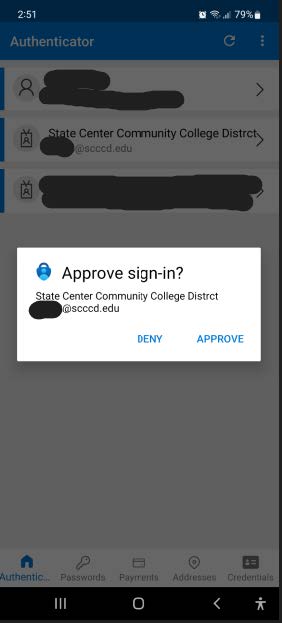A detailed image description of a smartphone screen displays a pop-up authentication prompt overlaying the background. Centrally on the screen, there's a prominent white rectangle with a light blue and blue icon on the left side. The main text within the rectangle reads, "Approve sign-in?" in bold black print. Directly beneath, in smaller text, it states, "State Center Community College District."

Under this header, a portion of an email address is visible but obscured, showing "[Name]@accord.edu," with the name redacted. At the bottom right of the rectangle, there are two clickable options in blue font: "Deny" and "Approve."

Above this authentication prompt, the screen’s header identifies the app as "Authenticator." There are three areas marked with black scribbles, effectively redacting sensitive information. The first scribble is adjacent to an icon depicting a silhouette of a person, the second conceals the email address, and the third blackens out two entire lines near an "A" character.

The background of the phone screen is noticeably darker and blurred, directing focus towards the authentication window.